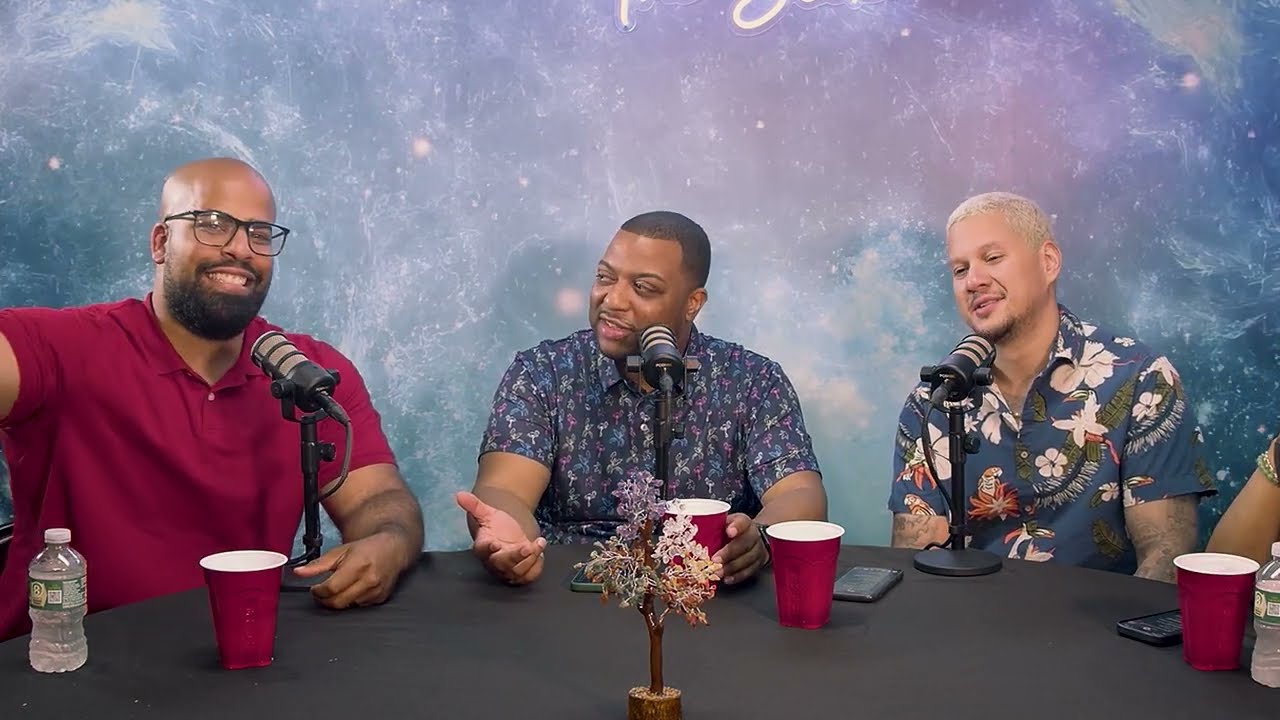In the image, three men are seated at a dark charcoal gray table participating in what appears to be a podcast or panel discussion. Microphones are positioned in front of them, suggesting a recorded conversation. The background features a mix of teal, purple, and lavender colors, adding a vibrant, almost night-sky effect to the setting.

On the far left sits a bald man with glasses and a short beard, dressed in a red, short-sleeved dress shirt. In front of him, there's a water bottle as well as a purple or magenta Solo cup, matching the cups each man has. The man in the center, who is black and has short dark hair, is wearing a dress shirt with floral designs and is looking to his right, engaged in dialogue. The man on the right stands out with his bleach blonde dyed hair, which contrasts with his natural facial hair, and he sports a blue Hawaiian shirt with white flowers and possibly bird images. His arms, showing tattoos, add to his distinctive appearance.

Additionally, a small tree sits at the center of the table, adding a touch of greenery to the scene. There is also someone slightly visible off to the side, likely a woman, partially hidden from the view. The overall setting appears carefully arranged, contributing to the podcast's inviting and colorful atmosphere.